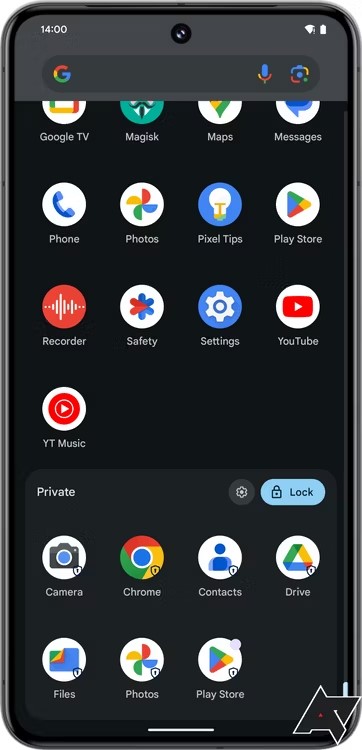A screenshot of a mobile phone homepage is captured, displaying a detailed glance at its interface at 14:00 hours. The Wi-Fi icon indicates connectivity issues, while the battery icon shows it is full or nearly full. Below the status bar, a Google search box is prominently placed. The wallpaper is a sleek, black background, enhancing the visibility of the various app icons. The screen showcases icons for Google TV, Magic, Maps, Messages, Phone, Photos, Pixel Tips, Play Store, Recorder, Safety, Settings, YouTube, and YouTube Music.

Further down the screen, there is a discreet white text that reads "Private" beside a lock button, allowing users to lock specific apps. Situated at the bottom are icons for Camera, Chrome, Contacts, Drive, Files, Photos, and Play Store, forming the primary app dock.